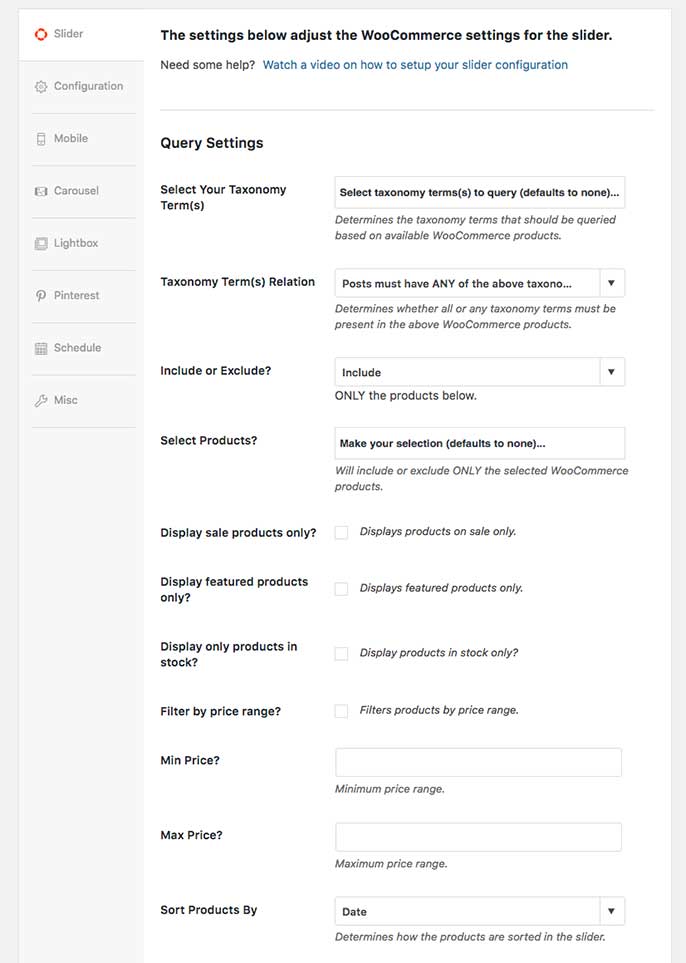This image showcases the settings page of a WooCommerce site specifically for configuring the slider. The page features a clean white background with bold black text for easy readability. At the top, a headline reads, "The settings below adjust the WooCommerce settings for the slider." The interface is primarily organized into various sections.

The "Query Settings" section is prominent, providing a dropdown menu for selecting taxonomy terms related to "relaxation." Users have the option to include or exclude specific terms or products within the slider. Another key section at the bottom offers "Filter Options," where users can filter products by price. This includes input boxes for defining the minimum and maximum price ranges. Additionally, there is an option to sort products by date, with inferred possibilities such as sorting by price also available.

On the left sidebar, multiple setting options are listed, including "Configuration," "Mobile," "Carousel," "Lightbox," "Pinterest," "Schedule," and "Miscellaneous." The current focus is on the "Slider" settings. Overall, this detailed settings page offers various customizable features to fine-tune the WooCommerce slider.